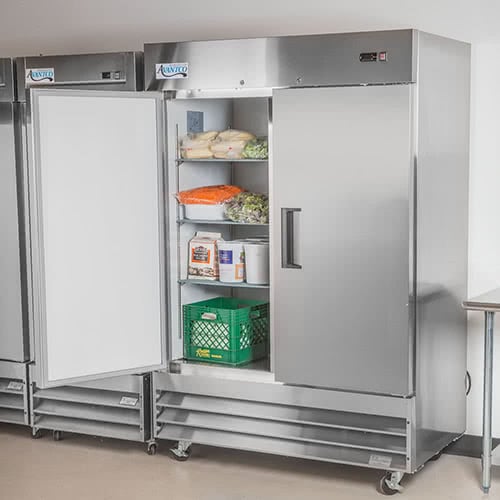The image depicts an industrial, silver, professional-grade refrigerator typical of a commercial kitchen, with a single door open on the left side. Inside the refrigerator are four shelves. The top shelf contains bags of rolls. The second shelf holds white plastic containers and an orange bag, possibly filled with vegetables, alongside a bag of green lettuce. On the third shelf sit more white containers. At the bottom, there's a green crate whose contents are not visible. The refrigerator is equipped with rollers for mobility and is situated on a beige marble-like floor. Adjacent to the right side of this refrigerator is a table with a metal frame, and to the left, another similar refrigerator unit is partially visible. The scene suggests a bustling kitchen environment, likely from a restaurant or diner.